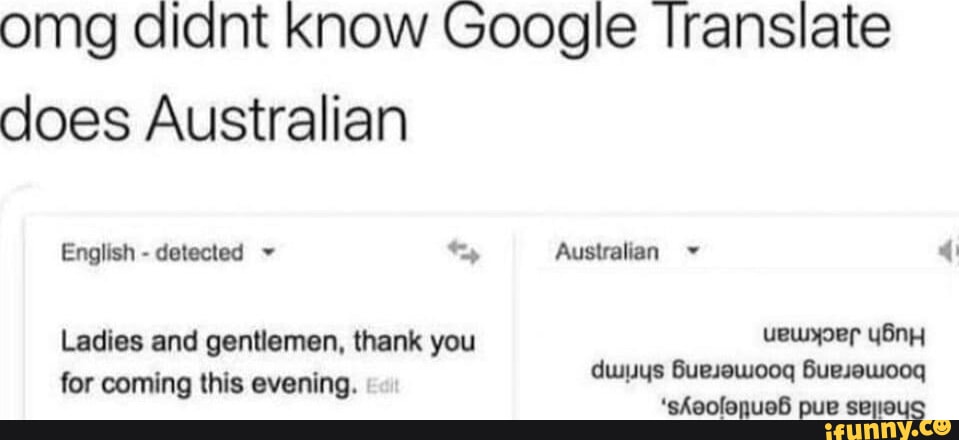Screenshot of a humorous meme, presented on an all-white background with a substantial amount of text. At the top of the image, prominently displayed in bold black letters, it reads: "OMG didn't know Google Translate does Australian." Below this text, there are two side-by-side translation boxes depicted, mimicking the Google Translate layout.

The first box on the left showcases the English translation interface. In the upper left corner of this box, it states "English detected" with a black drop-down arrow beside it, indicating the selection of the English language. The translation within this box reads: "Ladies and gentlemen, thank you for coming this evening."

Adjacent to this is the second translation box, representing the Australian version. At the top left of this box, it labels the language as "Australian" with an upside down black drop-down arrow, humorously suggesting the unique nature of Australian English. The content is implied to be an 'upside-down' version of the original English text, adding to the comedic effect.

At the very bottom of the image, there is a black banner stretching across the entire width of the screenshot. Positioned at the far right end of this banner is the text “iFunny.co.” Each letter in "iFunny.co" is yellow, and the letter "O" is stylized as a smiling face, indicating the source of the meme.